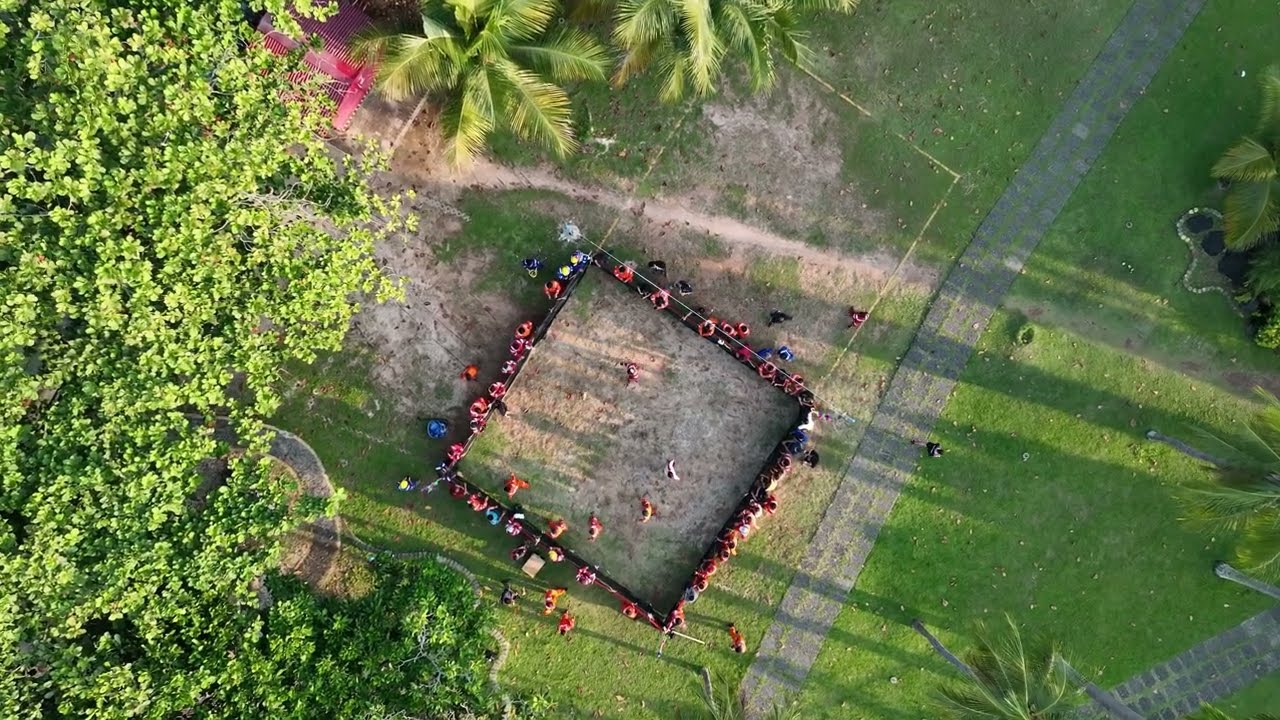In this detailed aerial view, a large square structure dominates a dry grassland area, surrounded by various vibrant elements. The grassland varies in color from green to dry patches. Bright green trees are visible to the left, while behind the square, palm trees dot the landscape. To the right of the square, there's a contrast between a lush, bright green lawn and more palm trees, with a paved gray path running through the scene. 

In the middle of the square, a cleared area hosts a gathering of people, some of whom are seated around the outside, suggesting a communal or social event possibly involving eating, while others appear to be walking inside. The square is festooned with items and flowers hanging from its walls, adding to the vibrant atmosphere. There's also something suggestive of animals—potentially roosters—within the square, hinting at a variety of activities.

Adjacent to the square, a narrow paved pathway cuts through the field, intersecting with another path that leads toward the top right of the image. Nearby, to the left, there's a circular concrete basin and more greenery with the tops of bamboo and other tree species visible. A pink item, possibly a tent, is located near the top left, adding a splash of color. Further to the right of the square, a line has been drawn on the ground, likely marking off another square or a designated playing area. This image captures a rich tapestry of human interaction and natural elements, all coalescing around the central square.